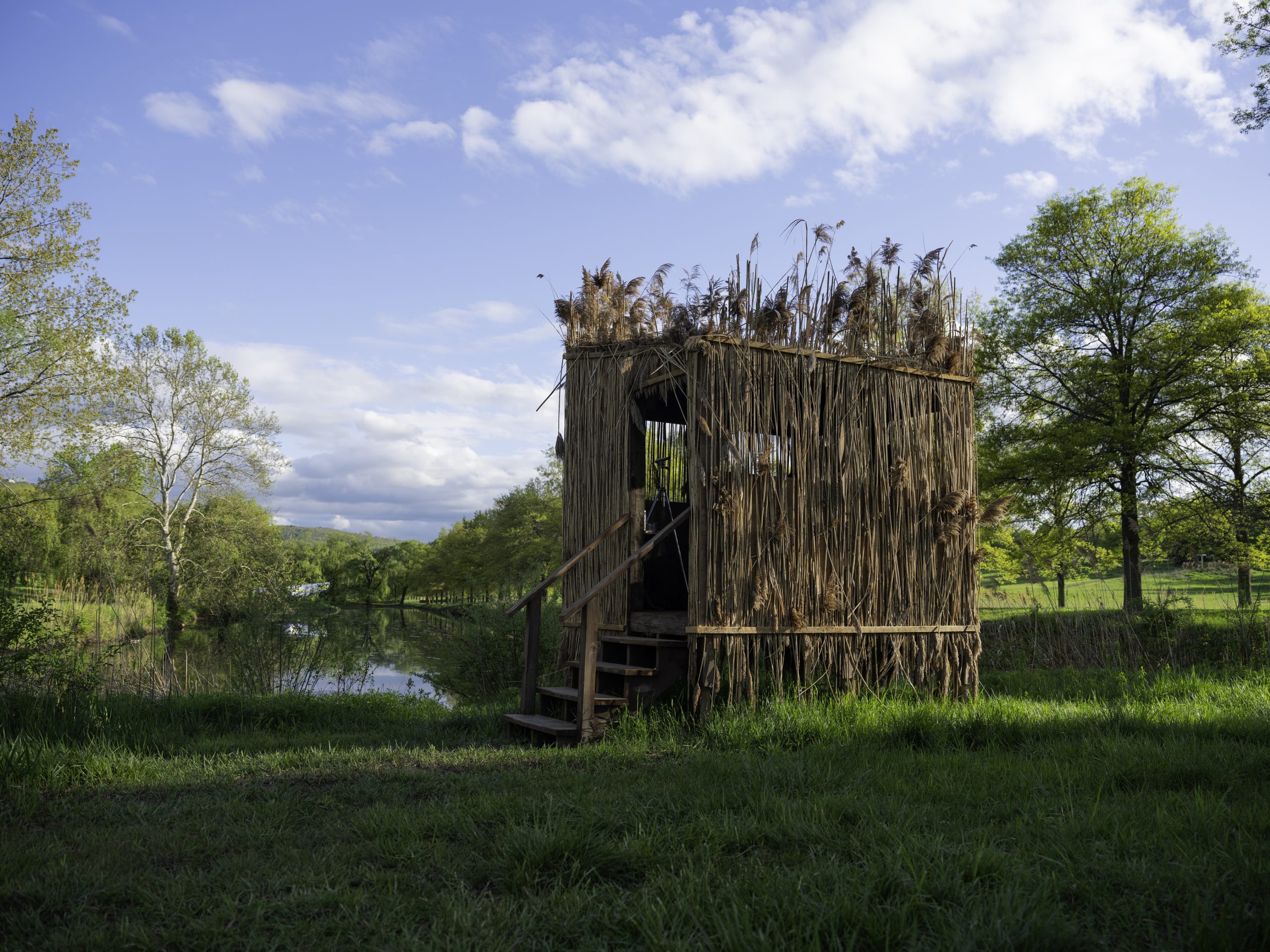Set in a serene, remote area with tall green grass, a small, calm pond, and surrounding trees, this scene features a rectangular, duck-hunting shack also suitable for birdwatching. Positioned right by the pond, this camouflaged structure is built from reeds that seem to blend seamlessly with its environment, resembling wheat or cotton-topped reeds from the pond itself. The shack is accessed via four wooden steps with hand railings leading to a small platform. The walls, framed with lumber, are thatched with reeds to enhance camouflage. Inside, visible through a square opening, the shack offers a vantage point for duck hunting or nature photography. The calm pond, dark in color and free of ripples, reflects the blue sky with scattered clouds, completing this tranquil, natural setting.